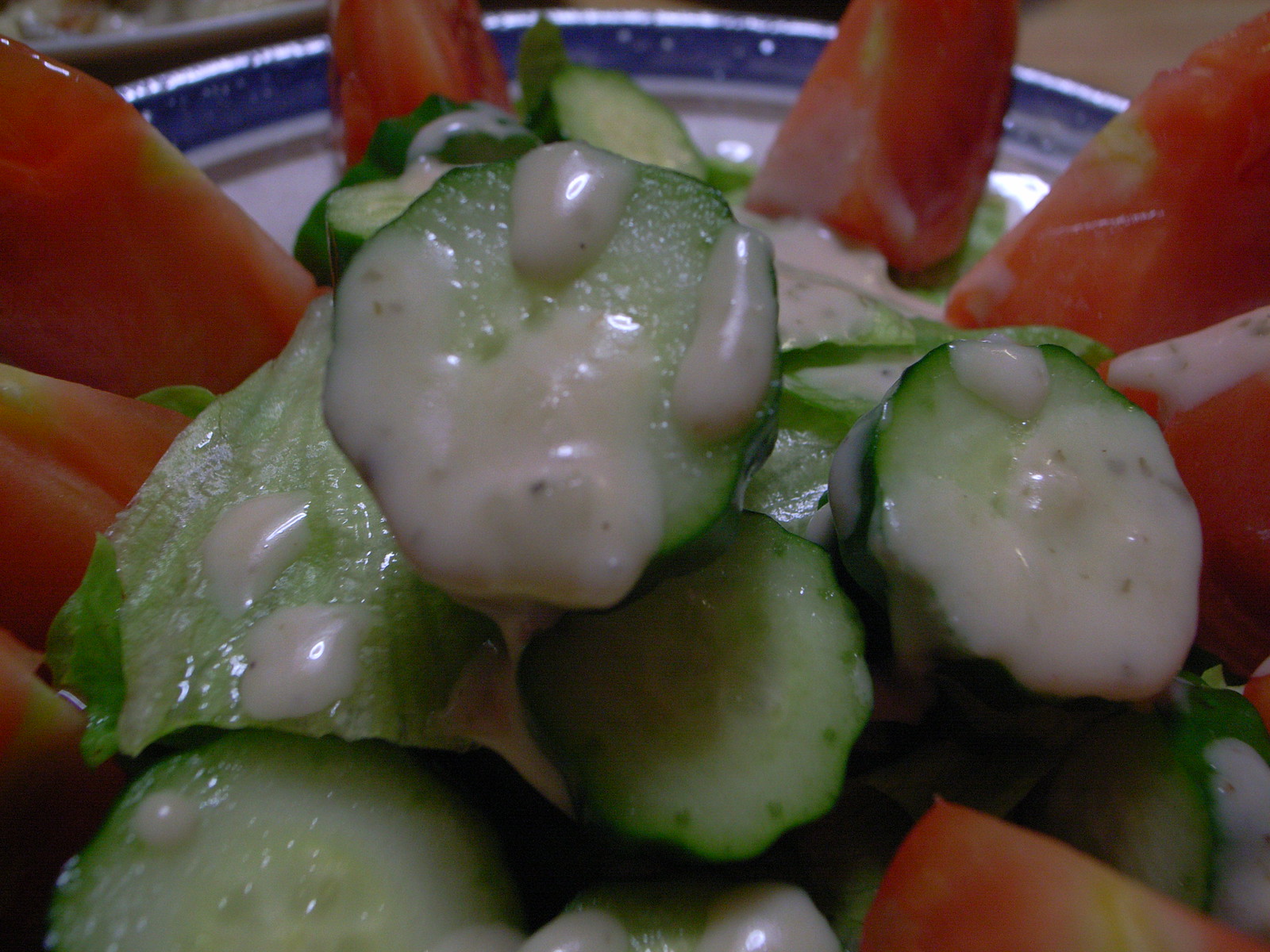The image portrays a vibrant salad artfully arranged on a white porcelain plate with a blue border. At the center, slices of fresh cucumber, cut crosswise, form the core of the dish, accentuated by a generous drizzle of creamy white ranch dressing, speckled with black flecks. Surrounding the cucumber slices, there are seven bright red tomato wedges, providing a striking contrast to the green cucumber. Although the cucumbers dominate the central area, there may be hints of green lettuce leaves interspersed within. The salad beautifully highlights the natural colors of the vegetables, with the green cucumbers in the middle and the red tomatoes around the edge, all presented on a circular, white plate with a distinct blue rim.